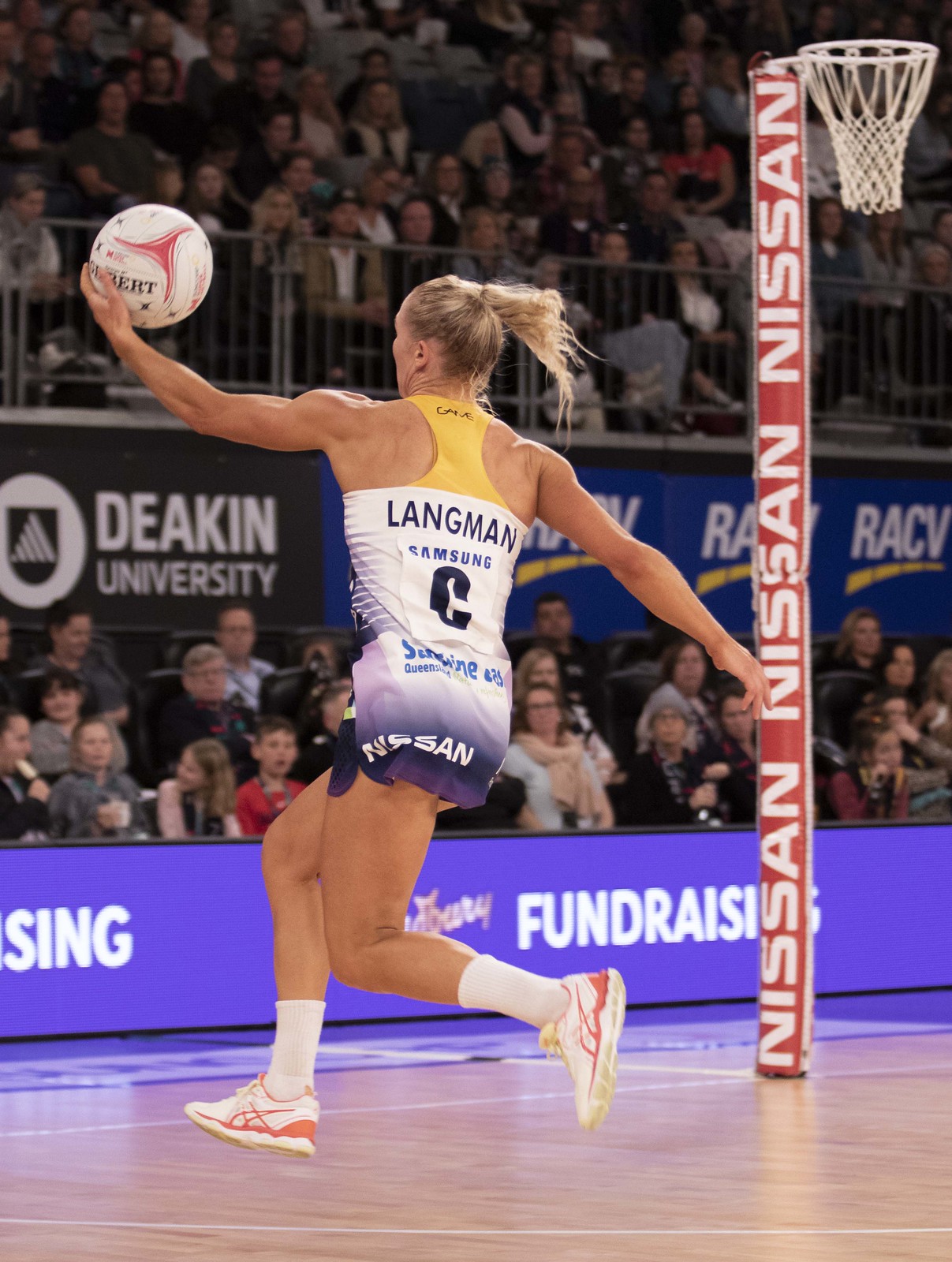A female volleyball player, with her blonde hair tied in a ponytail, stands on a wooden court, poised to serve the ball. She is seen from behind, wearing a distinctive yellow and white muscle-back tank top that has the name "Langman" along with "Samsung" and a large letter "C" printed on the back. Her outfit is completed with light and dark colored shorts and white shoes accented with apricot peach or tangerine tones. The volleyball in her hand is white with red designs and black text. In front of her, spectators are seated behind a purple barrier that has the word "fundraising" among other text. Behind her, a red and white basketball net with the word "Nissan" repeated three times vertically is visible. The gymnasium floor is marked with white lines, and additional sponsor banners are displayed, revealing more levels of spectators in the background.